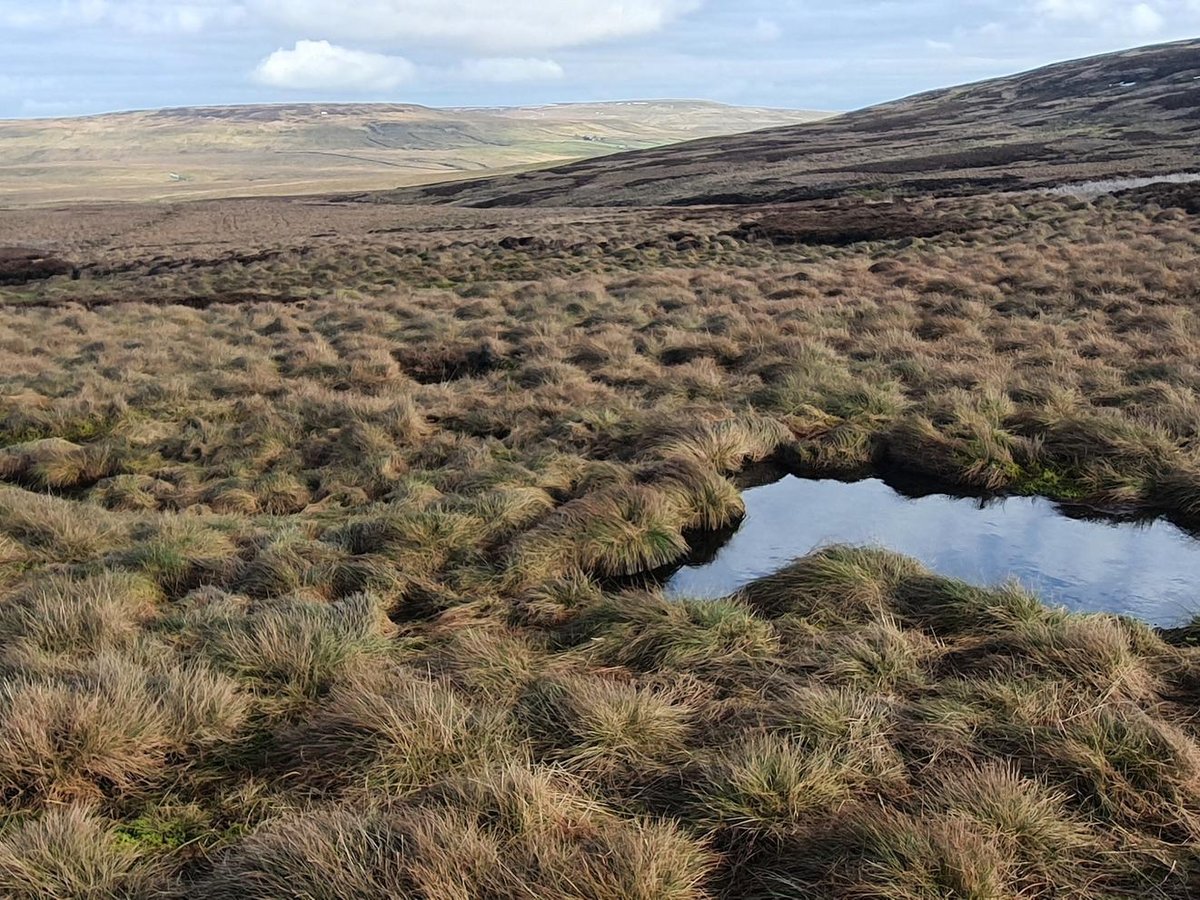The image captures a vast, desolate plain in stunning high quality. The distant horizon showcases a semi-blue sky adorned with scattered white clouds gently spreading across it. Rolling hills emerge in the midground, contributing to the landscape's arid and isolated appearance. Predominantly brown hues dominate the scene, with minimal evidence of animal life.

In the foreground, thick tufts of weed-like plants are dispersed throughout, characterized by spindly needles and leaves. These plants exhibit a greenish base, transitioning to a more brownish hue towards the tips, indicating they have dried out. Dominating the lower-right quadrant is a uniquely shaped puddle, resembling a boot with the toe pointing left. The puddle's surface reflects the blue sky above, adding a touch of color and serene beauty to the otherwise stark and barren terrain.